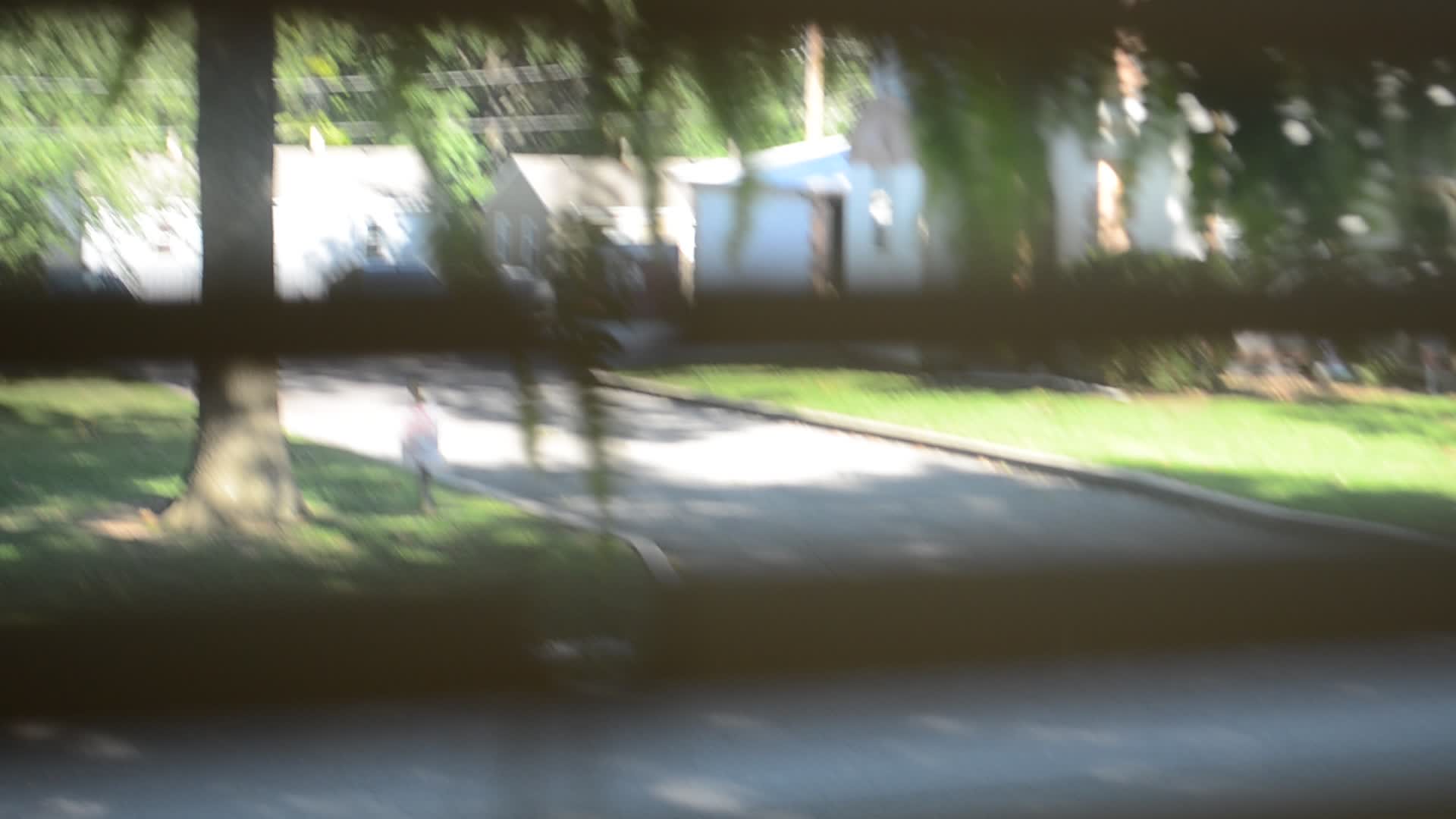This photograph, taken through window blinds, captures an outside neighborhood scene from within a home. The parallel dark lines of the blinds create an interesting overlay across the slightly blurry image. The photograph showcases a tranquil suburban road flanked by grass and curbs on both sides. On the far right, a series of whitish houses stand in a row, partially obscured by a cluster of trees and bushes. Dominating the left side of the image is a tall tree with a sturdy trunk and a canopy of branches and lush green leaves, creating an umbrella-like effect. Behind this tree, another house is visible, nestled among its neighboring homes. The overall ambiance of the photo suggests a serene, leafy neighborhood captured through the lens of domesticity.